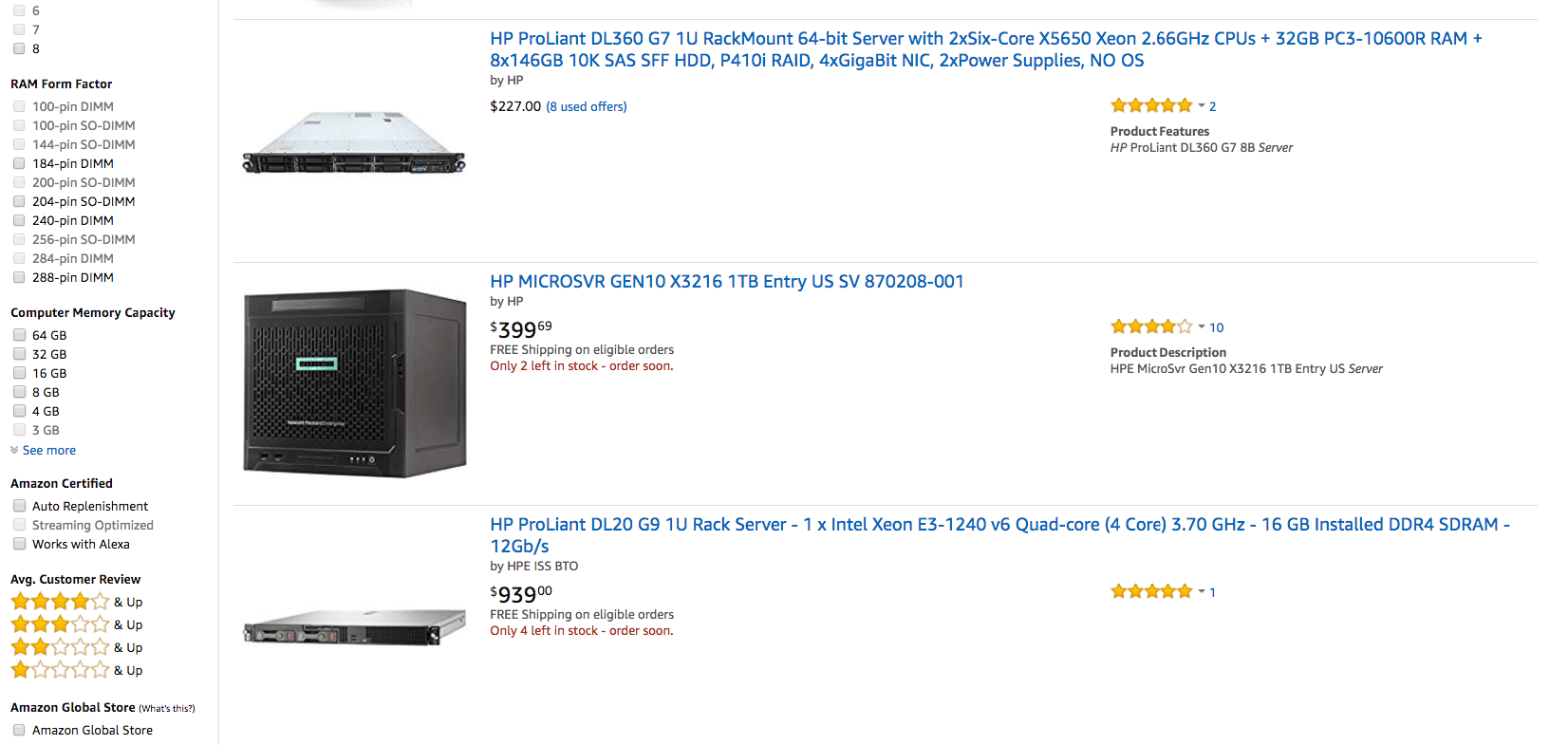This image showcases three distinct Amazon listings for HP servers. The first listing at the top features the HP ProLiant DL360 G7 1U Rack Mount server. This model is equipped with dual 6-core x55650 Xeon 2.66GHz CPUs, 32GB PC3 10600R RAM, and six 146GB 10K SAS SFF hard drives. The server has an impressive rating of 5 stars from 2 reviews.

The second listing displays the HP MicroServer Gen10 x32, priced at $399.69. This model comes with 16GB RAM and a 1TB hard drive, identified by the code SV870208-001. It has a rating of 4 stars based on 10 reviews and offers free shipping on qualifying orders. The listing also highlights that there are only 2 units left in stock, urging customers to order soon with a red warning.

The third listing is for the HP ProLiant DL20 G9 1U Rack Server. This server features an Intel Xeon E3 1240x6 Quad-Core processor running at 3.78GHz and includes 16GB DDR4 SD RAM. It is priced at $939 and also mentions free shipping on qualifying orders.